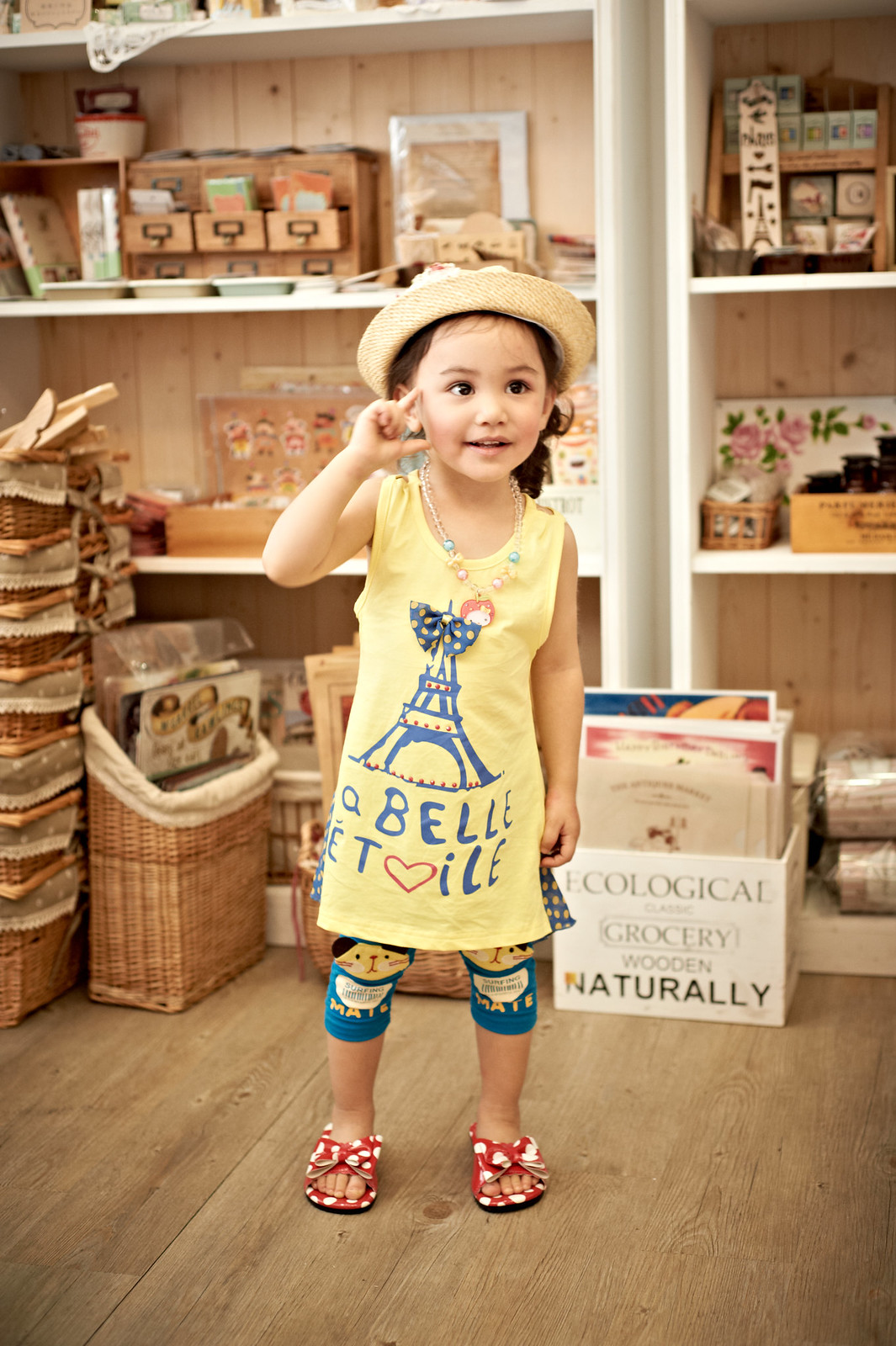In the photograph taken indoors, likely in a charming country store, a young girl stands centrally amidst a backdrop of rustic decor. She is adorned in a yellow tank top featuring an Eiffel Tower graphic with a bow, labeled "Belle Étoile." She pairs this with a straw hat and red and white slippers, appearing both relaxed and playful. Her right arm is raised with her index finger and thumb touching her cheek, while her left arm remains at her side. Behind her, white wooden shelves stocked with various items frame the scene, including a stack of wicker baskets lined with burlap in the left corner. Noteworthy is a small white crate labeled "Ecological Grocery Wooden Naturally" situated behind her left hip. The wooden plank flooring and the assortment of colors—brown, red, white, turquoise, tan, yellow, orange, red, green, pink—add to the quaint ambiance of the setting. The young girl gazes slightly to the right, capturing a moment of thoughtful stillness amidst the eclectic array of store items.